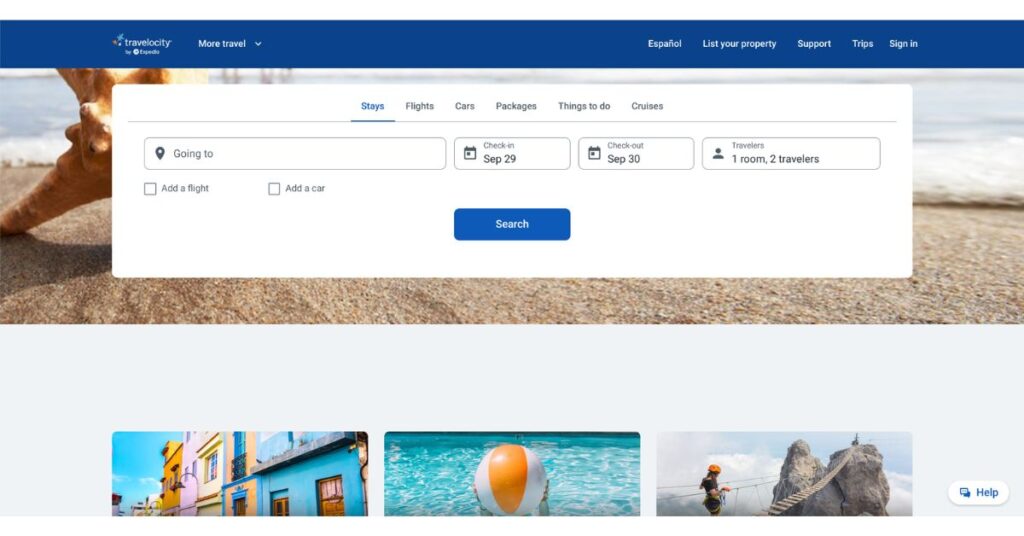This screenshot captures a partially cut-off webpage taken from a computer screen. The image is not in full vertical size, leaving some elements at the bottom cropped. At the top of the page, a blue border prominently displays the "Travelocity" logo on the left, followed by the text "More Travel" with a small drop-down caret. On the far right, also in white letters, are the options "Español," "List your property," "Support," "Trips," and "Sign in."

Beneath this navigation bar, a wide horizontal rectangle spans across the entire width, featuring an idyllic beach scene with a starfish by the shoreline. Overlaying this scenic background is a prominent white pop-up box that dominates the central area of the screen.

At the upper portion of this pop-up, several tabs are listed: "Stays," "Flights," "Cars," "Packages," "Things to do," and "Cruises." The "Stays" tab is highlighted in blue with a line underneath, indicating it is the selected option. Below this, there are fields for entering travel details, including destination, dates, and number of travelers, followed by a blue "Search" button.

Further down, a gray section includes three equally spaced images, though their bottom portions are cut off. The first image depicts vibrant, colorful houses, the second shows a swimming pool with a beach ball, and the third features a person hiking on a mountain.